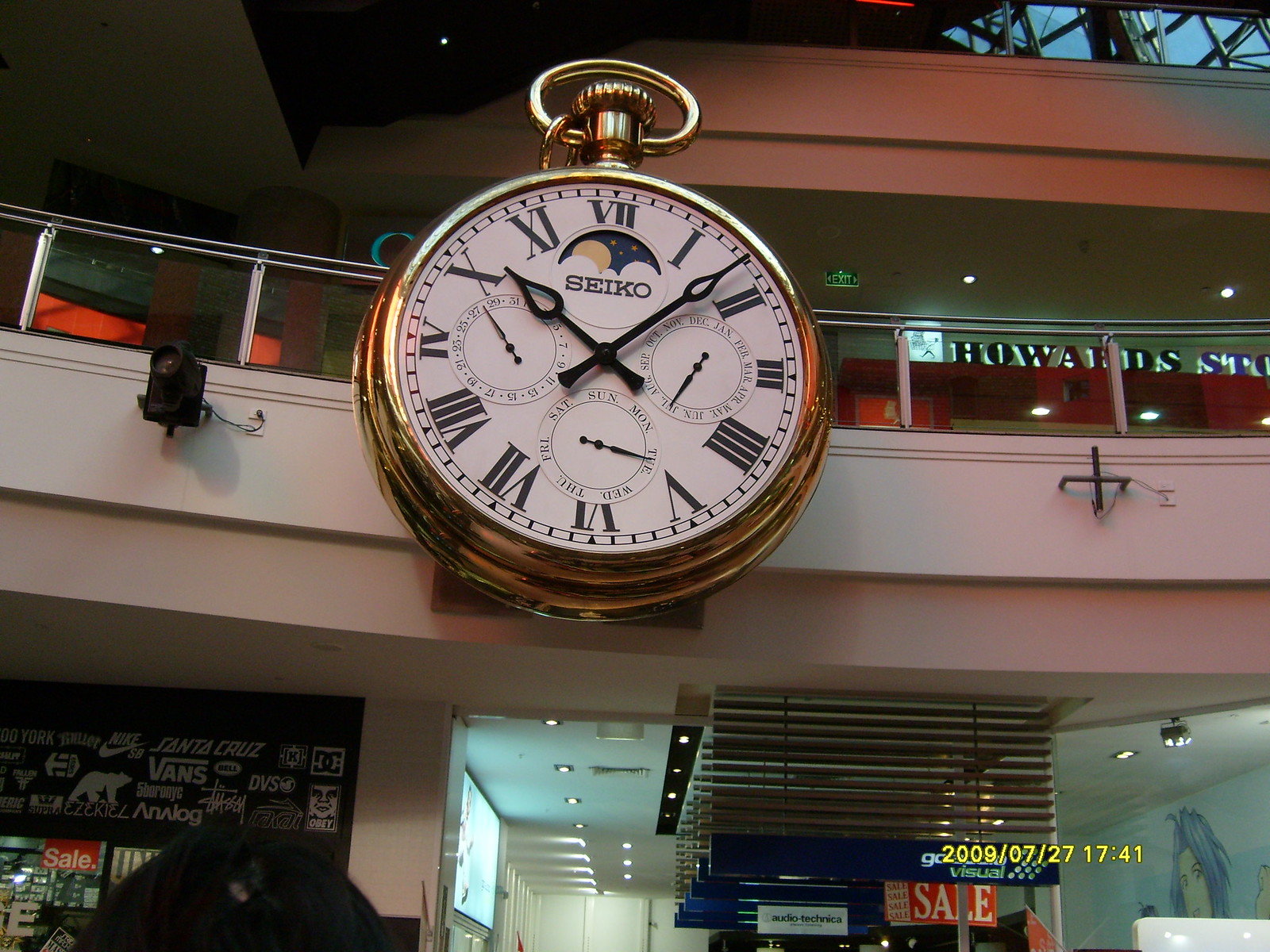The image showcases a large shopping center with an exterior predominantly painted in a soft pink hue, accented by a darker red color along the upper sections. A striking feature of the building is a massive, gold-colored clock designed to resemble an oversized pocket watch. The clock is prominently mounted on the wall and includes a visible chain loop at the top. The face of the clock is white, with bold black Roman numerals and black hands, and the brand name "Seiko" is printed in black letters at the center. Surrounding the shopping center is a modern glass fence, supported by pink poles that complement the building's primary color. Below the clock, various shops are visible, displaying ongoing sales. Notably, the timestamp "2009-07-27 at $17.41" is present, likely indicating the date and time the photo was taken.